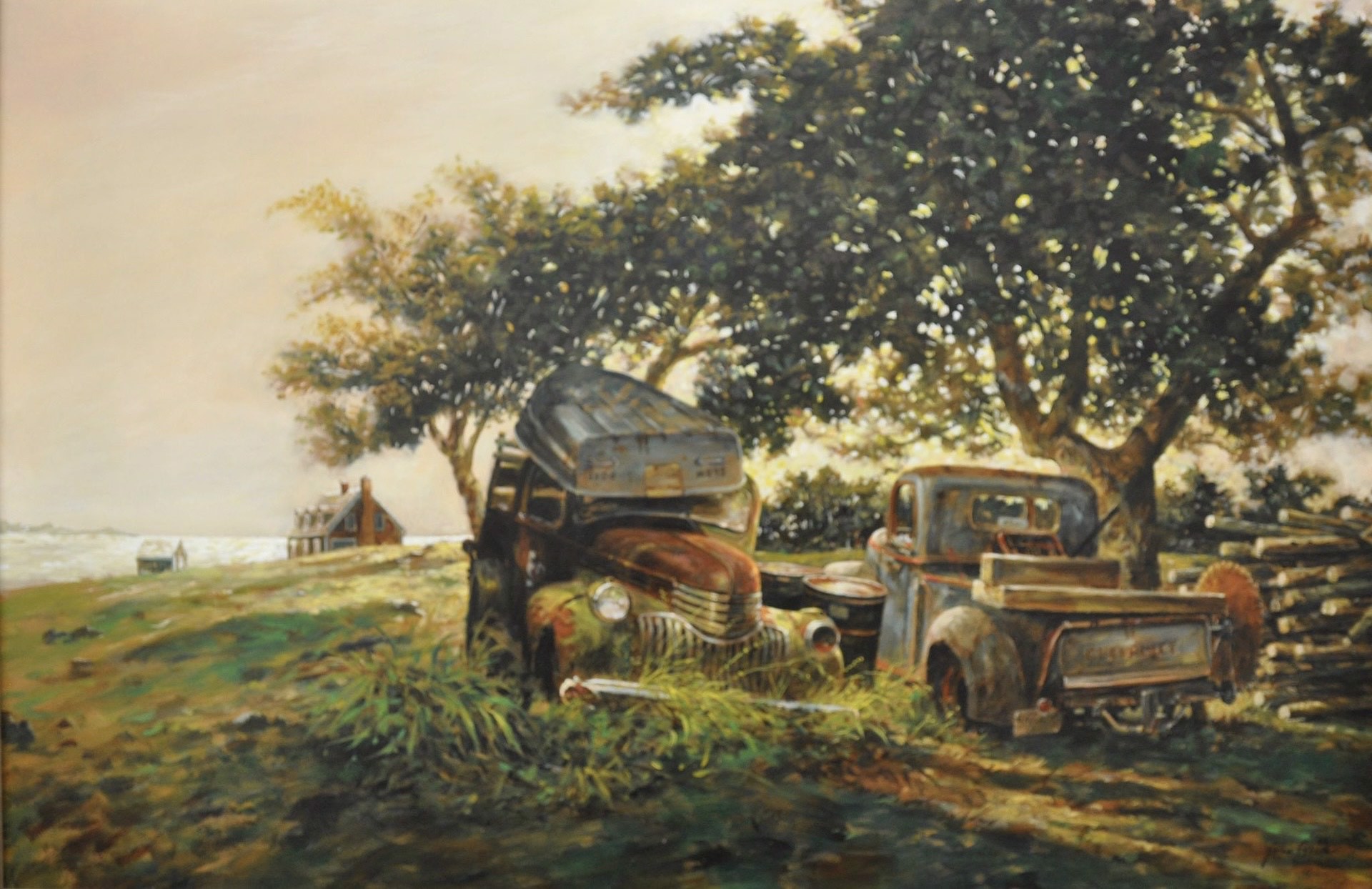The painting, which likely dates from within the last century, is a rich and vibrant depiction of a rustic country scene, possibly rendered in oil or acrylic. In the foreground, there are two old, possibly abandoned vehicles: a rusted pickup truck with a small metal boat on its roof and another vehicle that appears to be a station wagon. Both of these vehicles are surrounded by overgrown grass and weeds, emphasizing their state of neglect. To the right of the pickup truck, there is a pile of sod logs or lumber. The scene is dominated by natural elements, with a large oak tree standing prominently behind the vehicles. The background features a sloping hillside dotted with more trees, leading down to an old farmhouse and a small barn situated near a shoreline, suggesting the presence of water like an ocean in the far distance. The sky overhead is overcast, adding to the painting's rustic and slightly somber atmosphere.